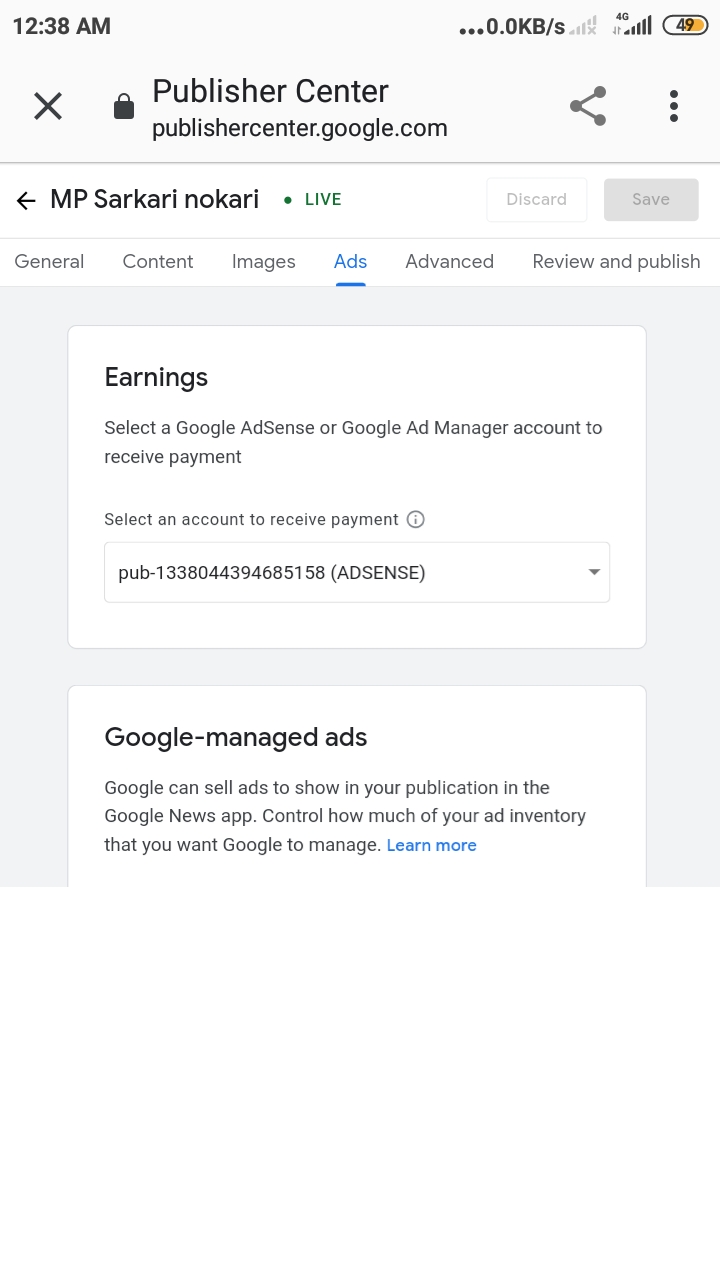A screenshot from a smartphone displaying an interface from the Google Publisher Center (publishercenter.google.com). At the top of the screen, the logged-in user is identified as "MP Sakari Nokari," accompanied by a green "live" indicator with a dot. Below this, there are six navigation tabs labeled: General, Content, Images, Ads, Advanced, Review and Publish, with the "Ads" tab currently selected.

The highlighted "Ads" section shows options for managing earnings. It prompts the user to select a Google AdSense or Google Ad Manager account to receive payment, and a drop-down menu is visible with one of the accounts selected. Further down, a section titled "Google Managed Ads" appears, explaining that Google can sell ads to display in the user's publication within the Google News app, and offers control over the portion of ad inventory Google will manage.

The phone's time is displayed at the top left corner as 12:38 a.m., and the top right corner shows the battery status, which is currently at 49% and charging.